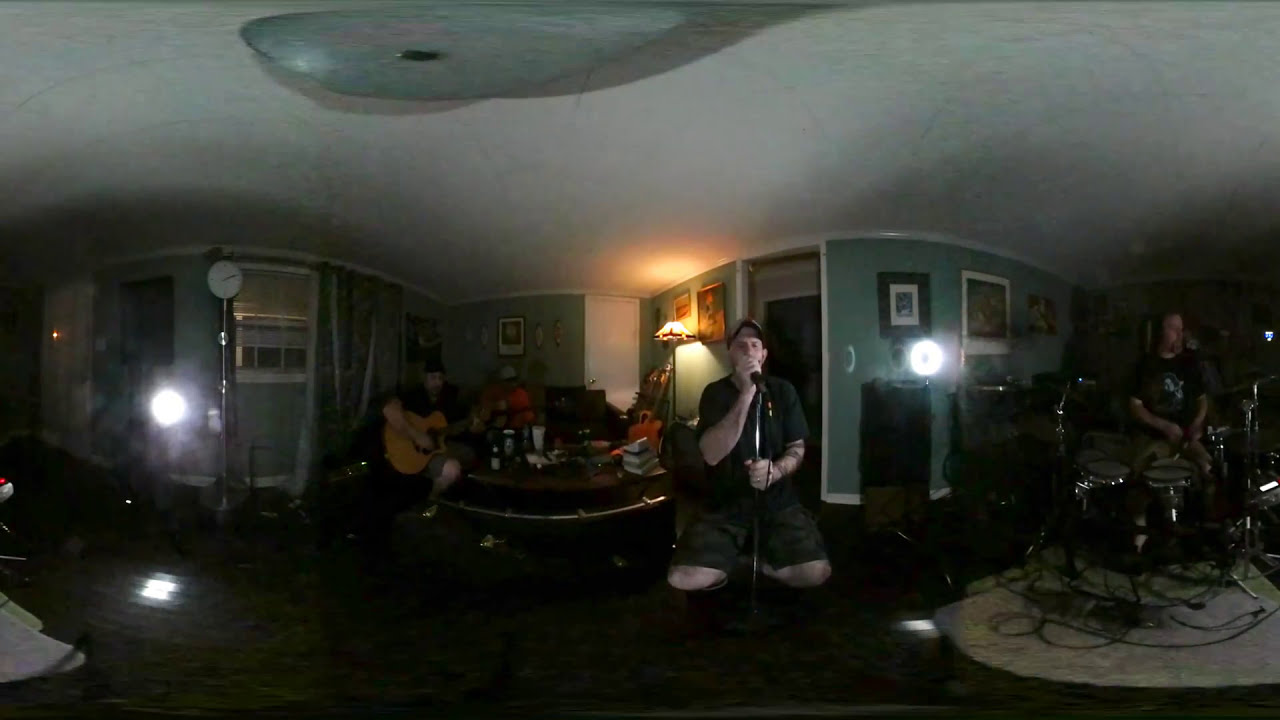The image depicts a home-based band performance captured with a 360-degree camera, resulting in a warped, curved appearance. The setting is an indoor living room with sage green walls adorned with picture frames and paintings. The white ceiling contrasts with the dark brown plank or hardwood flooring. 

In the middle of the room, a singer sits on a chair, clad in a black T-shirt, green cargo shorts, and a baseball cap, gripping a microphone and its stand. To his left, two musicians are strumming acoustic guitars, seated on a couch with a coffee table in front of them, loaded with books and water bottles. On the right side of the image is a drummer playing a black drum set, positioned on a white carpet. The room's windows have white shutters or blinds, and there are ring lights behind the drummer adding ambiance to the somewhat dark room; likely, they are setting up for an online recording or live stream. The overall room decor and lighting, combined with the musical setup, create an intimate and detailed atmosphere.